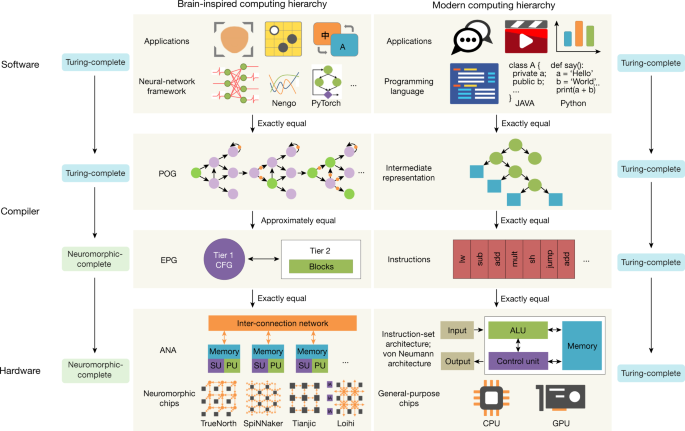This image appears to be a slide from a presentation, featuring multiple charts and diagrams. On the left side, there is a series of visual aids illustrating the hierarchy of brain-inspired computing, which includes charts related to software and computer hardware. These diagrams elaborate on various components and levels of brain-inspired computational systems. Adjacent to these, in a separate column, a modern computer computing hierarchy is depicted with its own set of charts. Finally, on the right-hand side of the slide, there is a recurring chart labeled "Turing Complete," reflecting a concept from computational theory that denotes systems capable of performing any computation, given enough resources. The detailed comparative visuals aim to delineate the differences and parallels between advanced computational paradigms.